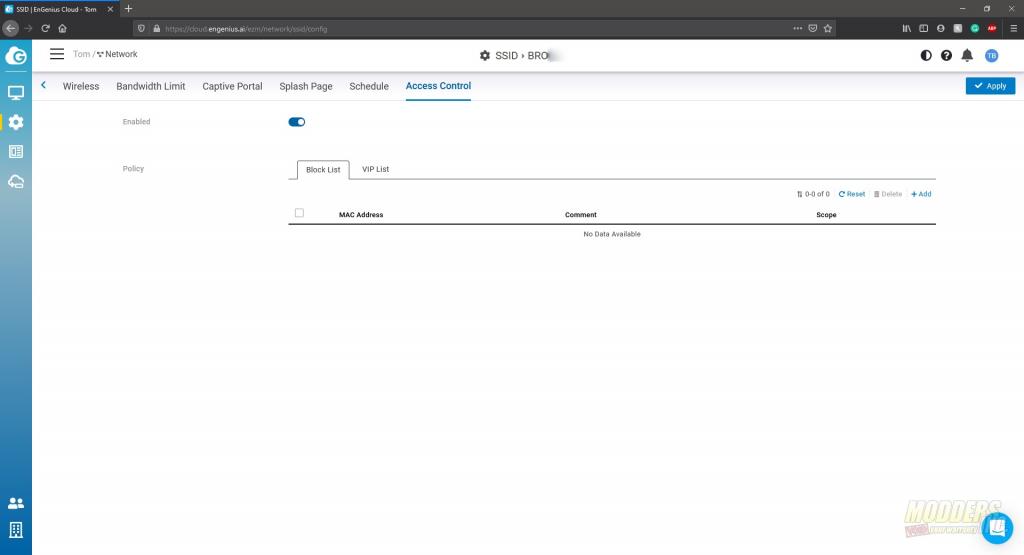The image depicts a detailed user interface for an SSD (Solid-State Drive) management tool with various network and cloud integration features. 

At the top, the interface title "SSD EN Ingenious Cloud Tab" is prominently displayed. Below it, there's a section where users can add an additional tab. 

The left side of the interface shows a search bar and the website from which this tool is accessed. Adjacent to the left arrow is a "gcloud" icon, featuring a stylized "g" with a cloud graphic.

Below this, several icons are illustrated including a computer monitor, a gearbox, what appears to be a TV symbol, another cloud, and a three-line menu commonly known as a hamburger menu. These icons are labeled with terms such as "tab," "splash," and "network."

Further down, additional functionalities are listed: "wireless," page navigation, a bandwidth limit configuration, a captive portal, and a splash page schedule. The "access control" section is highlighted in blue, indicating the current page being shown, with a horizontal line beneath it. On the far right, there is an "apply" button within a block.

Above the "apply" button are contrast adjustment icons, a question mark for help, an alert icon, and a current status indicator labeled "TV" in blue. Below the bandwidth information, there is an "enabled" slider button to toggle the feature on or off.

In the same row as the enabled button, there are columns labeled "Policy" and "Block List," featuring a checkbox for "MAC address" (currently unselected). Next to this is a "VIP List" tab.

The overall layout is intricate, providing comprehensive control and visualization options for the SSD management tool, emphasizing cloud and network functionality.